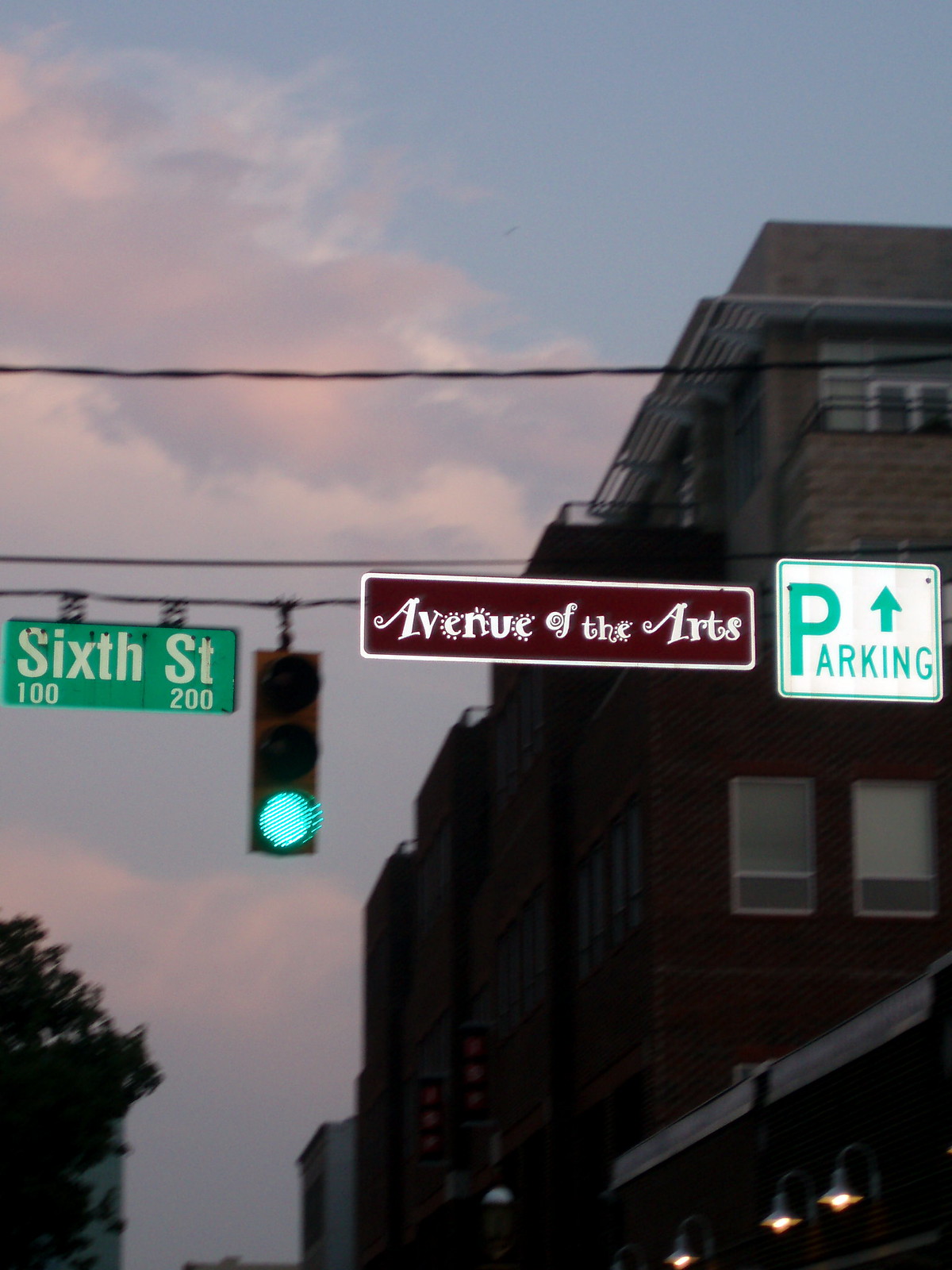The photograph captures a street scene at dusk, featuring an array of street signs and a traffic light suspended above an intersection by cables. Dominating the scene is a set of three distinct signs: the leftmost sign is green with white text, marking "6th Street" between 100 and 200; the central sign is red with a white border and stylized white text that reads "Avenue of the Arts"; and the rightmost sign is white bordered by green, displaying "Parking" in green text with an upward-pointing arrow. Behind these signs, a traffic light shows green, indicating proceed. The backdrop includes a tall brown brick building with numerous windows and balconies, partially obscured by a dim, blue sky that hints at the coming night, accented by streaks of white and purple clouds. This scene, likely pictured at a 45-degree angle from someone in a car or on the street, captures the atmosphere and architectural elements typical of a busy urban intersection.